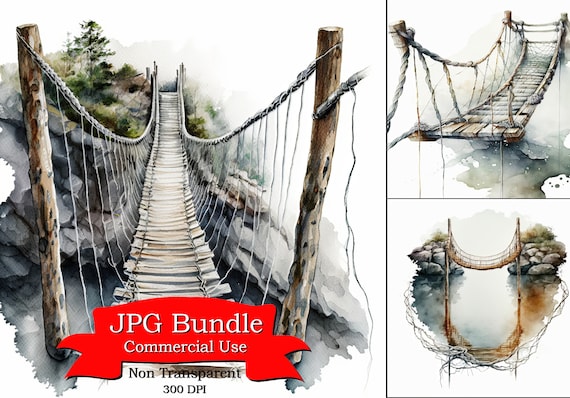This is a detailed watercolor drawing of a rickety swinging bridge made of wooden beams and ropes, extending over a rocky, water-filled area. The bridge is depicted in shades of brown and gray, with mountainous terrain and green trees visible in the blurred background. The sky is painted a soft blue. In the forefront of the image, a red ribbon with white text reads "JPG bundle commercial use," and just below it, in black text, it states "non-transparent 300 DPI." To the right of the main image, there are two additional pictures. The first provides a close-up view, highlighting the bridge's rope sides and wooden planks. The second offers a distant perspective, showcasing the entire bridge spanning from left to right between two rocky hills with the white, gray, and brown water beneath it.